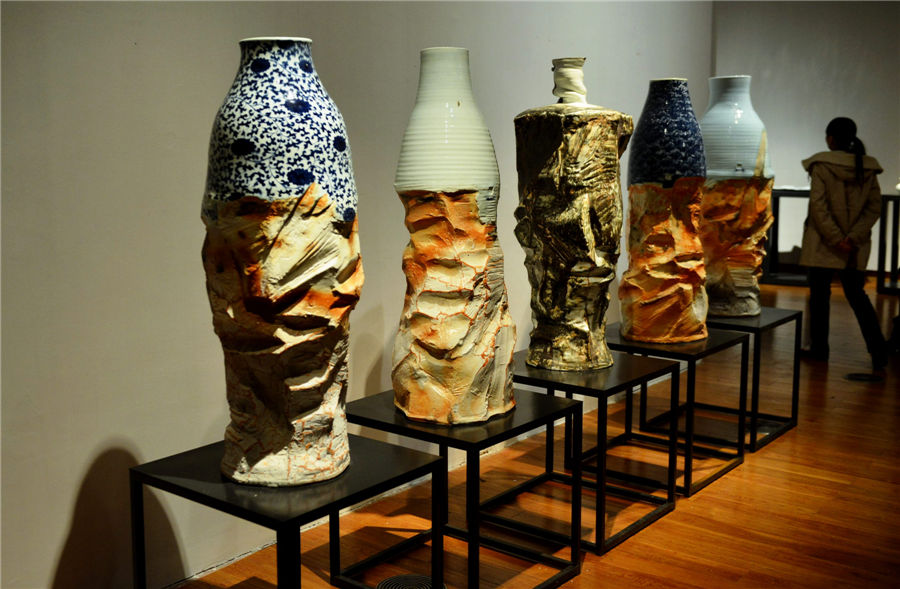This is a detailed color photograph capturing the interior of an art gallery or museum. The central focus is a row of five large vases, each uniquely crafted with various glazes in different colors, sizes, and shapes. These modern art pieces are intriguingly mounted on chiseled stone holders that have a white and reddish-brown hue, and they rest atop sleek black table stands. The vases are lined up against a plain white wall and are arranged in a diagonal from the lower left to the middle right of the image. One vase is predominantly blue and white, another is mostly white, the central one is smaller and cylindrical, followed by a cobalt blue vase, and the last one is mainly white. Illuminated by ceiling-mounted track lighting, the scene is set on a dark brown hardwood floor. In the background, a spectator dressed in a jacket stands in the upper right corner, observing other artworks with hands behind her back.